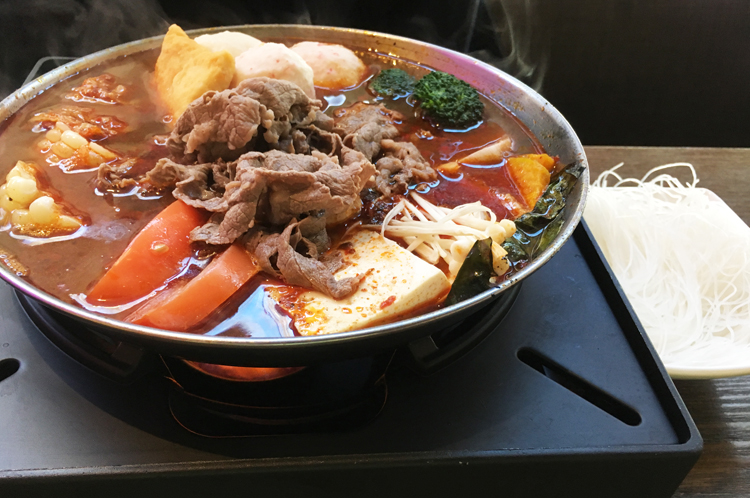This image captures a simmering bowl of ramen on an individual burner, set against a black background, possibly a black wall or backdrop, all on a wooden table. The ramen is housed in a large metal bowl placed on a black square base resembling a stove, with steam visibly rising, indicating the dish's hot temperature. At the center of the bowl lies thinly sliced beef, immersed in a warm, rich brown broth. The broth is generously garnished with an array of vegetables and other ingredients: delicate thin noodles, vibrant green broccoli florets, and cooked leafy greens. Scattered around are slices of carrot, chunks of tofu, and pieces of corn on the cob. On the table to the right of the burner, a white rectangular dish holds uncooked, very thin, delicate noodles, providing a contrast to the hot, steaming ramen. The scene evokes a sense of warmth and comfort, ready for a savory meal.